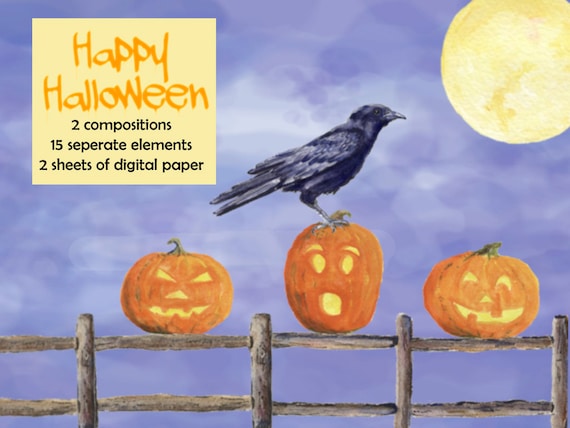The image depicts a Halloween-themed digital composition that resembles packaging for postcards or holiday cards. Central to the scene is a simple wooden fence adorned with three carved jack-o'-lanterns. The middle pumpkin, with a shocked expression, is the tallest and serves as a perch for a raven facing to the right. The sky forms a dramatic backdrop with a purplish hue, evocative of an evening dusk, and features a large, yellowish moon in the upper right corner. In the upper left, a yellow box with ornate orange lettering reads "Happy Halloween," with black text underneath listing "two compositions, fifteen separate elements, two sheets of digital paper." The combined elements of the wooden fence, the trio of expressive jack-o'-lanterns, the perched raven, and the haunting twilight sky come together to create a vivid and detailed Halloween scene.